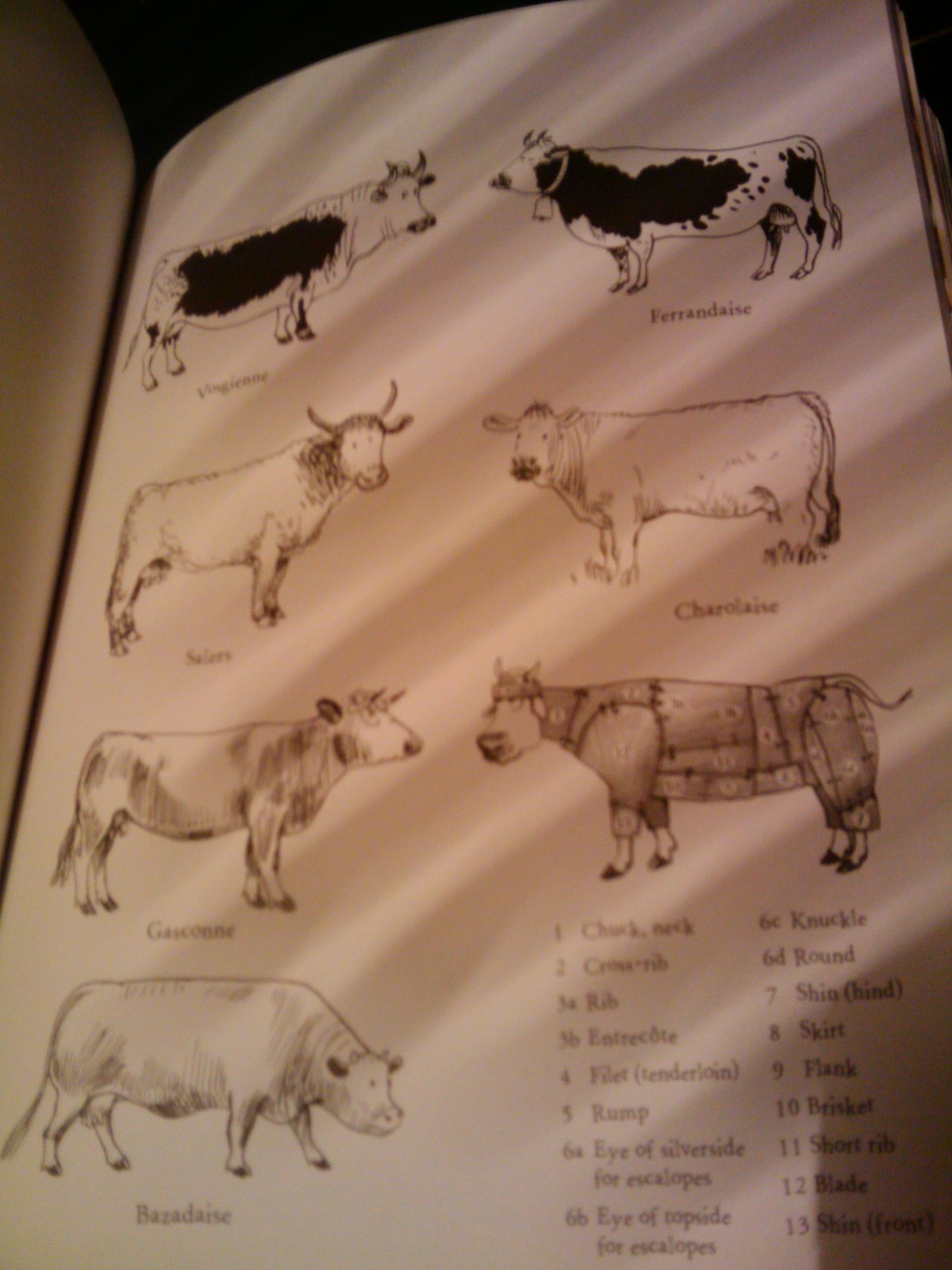This is a detailed photograph from a French textbook or encyclopedia showcasing various breeds of cattle and their butchering parts. The image displays seven illustrations of different cows and bulls arranged in two rows of three, with one additional image on the bottom left. The cows vary in shapes and sizes but are distinctly recognizable. Labels beneath each cow denote their breed names, although the text is somewhat blurry. Identifiable breeds include one starting with a "V" that's primarily white with a large black splotch, another facing it, Ferrandes (with black closer to the front), Charelais, and Gascogne. The lower left corner features Bazardes.

On the lower right, there's a detailed diagram of a cow marked with various sections, resembling wood panels with numbered areas from 1 to 13, with detailed subsections labeled 6A, 6B, 6C, and 6D. This diagram correlates to a list of butchering cuts, including chuck neck, cross rib, rib, intercostal, fillet, rump, silver side, top side, knuckle, round, shin, hind, skirt, flank, brisket, short rib, blade, and shin front. This informative layout clearly indicates where each cut of meat is located on the cow.